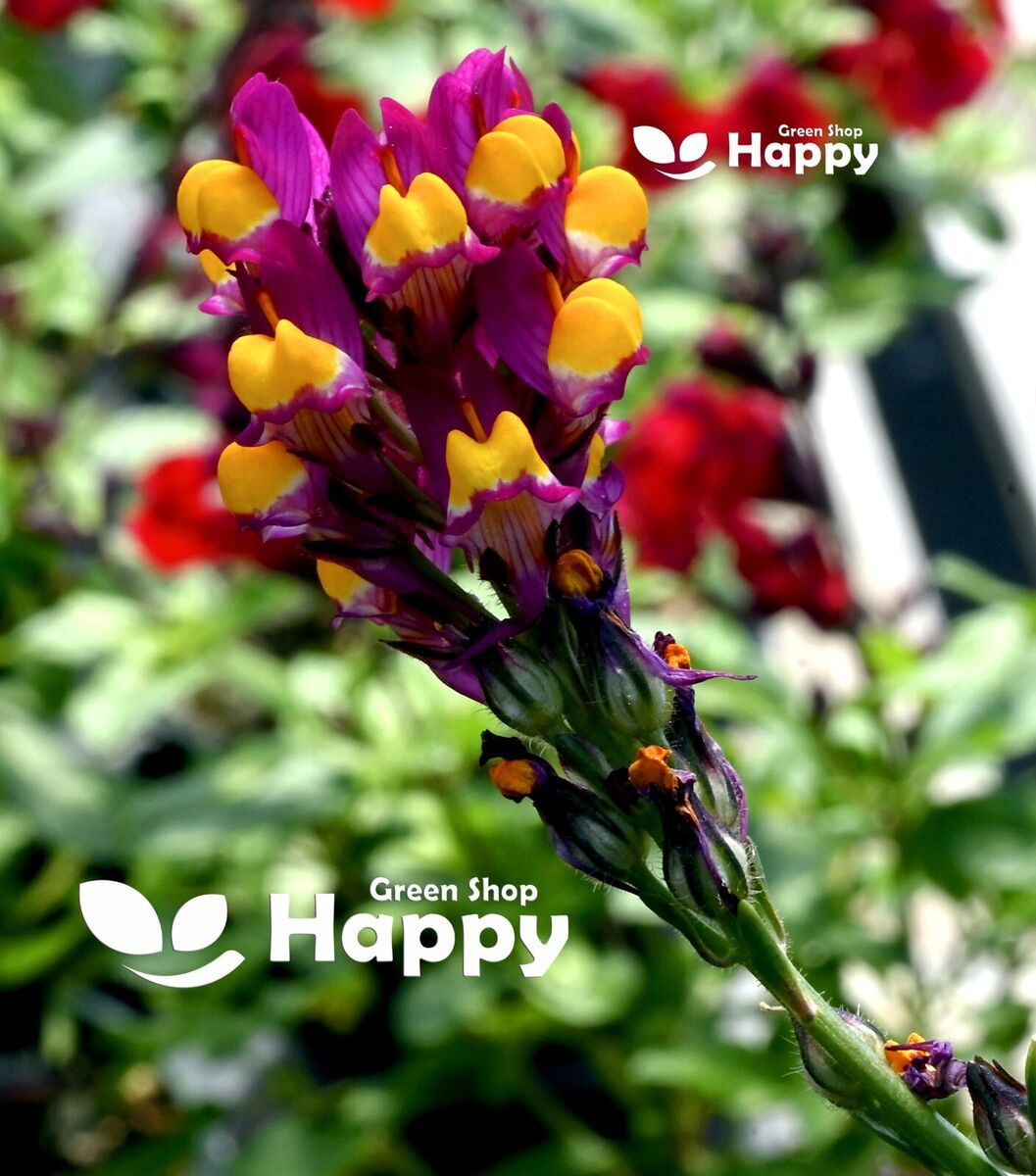This square, close-up color image centers on a bouquet of flowers dominated by delicate, purple petals and vibrant yellow centers, possibly snapdragons or orchids. The green stems have a slight fuzz of tiny spikes. Blossoming flowers branch upward towards the upper left corner, while some are poised to bloom near the bottom. The out-of-focus background consists of lush green foliage interspersed with red flowers, emphasizing the bouquet. White text in the top right and bottom left corners reads "Green Shop Happy," each accompanied by a logo featuring white leaves and a curved shape. The blurred backdrop ensures the viewer's attention remains on the intricate details of the vibrant flowers in the foreground.